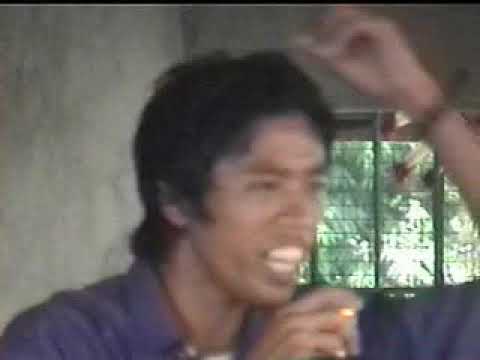The image captures an Asian man, possibly Indonesian or Filipino, with brown skin and a big smile showcasing his white teeth. He has medium-length black hair and is wearing a blue collared shirt over a white undershirt. His appearance suggests he might be conversing enthusiastically, as his mouth is open and his arms are animated in gestures. A watch adorns his left wrist. The room where he stands features grey and brown walls, and a window with blinds. Through the blinds, green trees are visible against the sunlight. The overall quality of the image is somewhat blurred, giving it the appearance of a video screenshot.